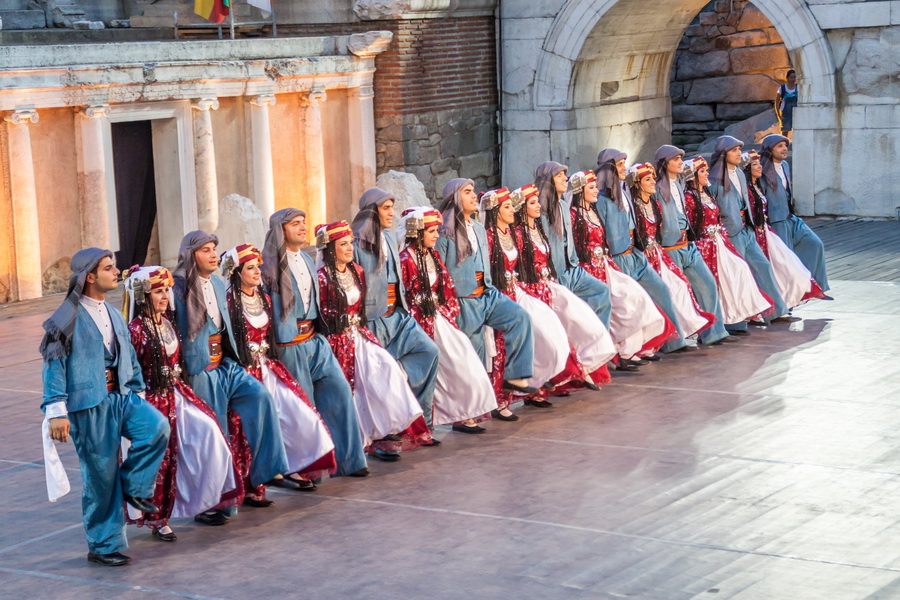The image captures a lively scene of men and women in traditional attire performing a cultural dance in front of a historical building. The dancers are arranged in a diagonal line from the bottom left to the top right of the frame, alternating between men and women, with the center featuring two women. The men are dressed in blue jackets with loose blue pants, white button-up shirts underneath, and blue head coverings, while the women wear elegant red dresses with white underlayers, accompanied by white head coverings adorned with red and yellow accents. Each dancer raises their left knee and engages with the dynamic movements of the dance. The background showcases a historical setting with a stone entryway in the top right, complete with a visible onlooker dressed in distinctive attire peering through the arch. Additionally, white pillars and part of a brick wall on the left side enhance the architectural depth. The scene is vibrant with vivid colors, including blue, orange, red, white, gray, tan, and yellow, contributing to the rich cultural tapestry depicted in the photo.